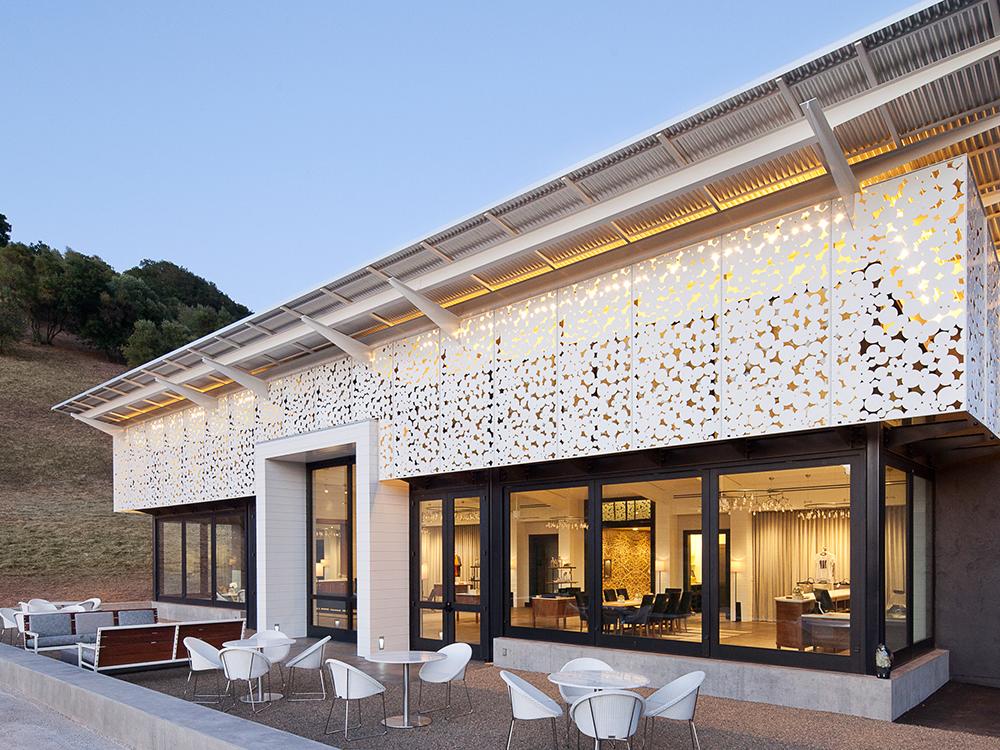The image depicts a strikingly modern restaurant nestled in an open field, characterized by its sleek white design. Dominating the structure are large, black-framed windows that provide an expansive view of the luxurious interior. The roof is an eye-catching feature with its curved, corrugated metal that adds to the contemporary aesthetic. Inside, the restaurant exudes an elegant ambiance with golden and brown tones, accentuated by lavish lighting and very large, see-through windows.

The restaurant features various dining areas, including a main area with multiple dining tables surrounded by chic, blue chairs. There seems to be a bar situated on the right side. The outside patio area, paved with concrete, continues the sophisticated theme. Circular tables with white tops are encircled by unique, conical-shaped chairs. A wooden bench with blue cushions provides additional seating on the left side of the patio.

The surrounding landscape highlights a large hill with neatly cut grass on one side and a scattering of trees at the top, set against a backdrop of a pristine, baby blue sky. The combination of the modern structure, the elegant interior, and the serene natural setting creates an inviting and visually appealing dining experience.